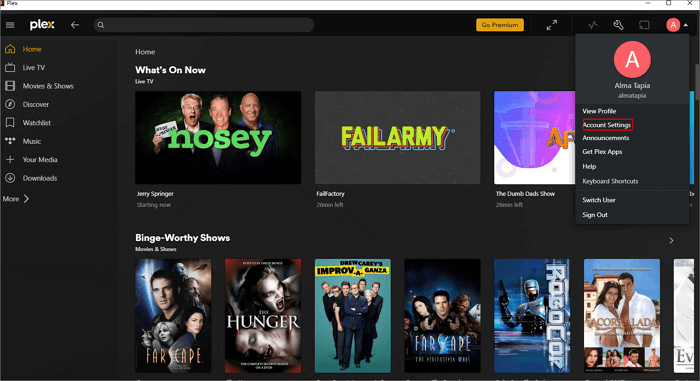The image depicts a webpage interface for the streaming service Plex, which offers movies, TV shows, and other media content. 

**Top Section:**
- **Logo:** In the top left corner, the Plex logo is prominently displayed. The letters "P L E" are in white, and the "X" is a blend of orange and white.
- **Hamburger Menu:** To the left of the logo, there is a hamburger menu icon.
- **Search Bar:** The search bar is positioned to the right of the Plex logo. The search bar is currently empty and features a white magnifying glass icon on the far left.
- **User Profile and Icons:** At the top right, there is a user profile icon represented by a red circle with the letter "A" in the center. Adjacent to the profile icon, from left to right, are the screen share icon, wrench icon (likely for settings), and expand icon. Additionally, there is an orange rectangular box with the words "Go Premium" centered within it.

**Left Sidebar:**
- **Categories:** Below the Plex logo, a vertical sidebar lists various navigation categories:
  - Home
  - Live TV
  - Movies & Shows
  - Discover
  - Watchlist
  - Music
  - Your Media
  - Downloads
- **More Section:** At the bottom of the sidebar, there is a "More" section with an arrow pointing to the right.

**Main Content Section:**
- **Header:** In the middle left portion of the image, the header reads, "What's On Now?"
- **Current Shows:** Below this header, several show titles are listed, including Jerry Springer, Fall Factory, and The Dumb Dumb Show.

Overall, the screenshot provides a comprehensive view of the Plex interface, showcasing its navigation tools, user options, and currently available content.